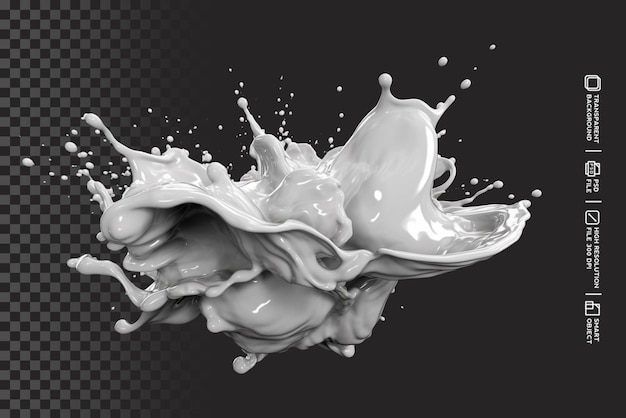This hyper-realistic black and white digital illustration captures a mesmerizing splash of white liquid, caught in mid-air with droplets and sheets of fluid spreading outward from a central blob. The shimmering liquid, rendered with exceptional detail, features intricate shadows that enhance its lifelike appearance. The background transitions from a black and gray checkerboard pattern on the left to a plain dark black on the right. Vertically aligned on the right-hand side, white text reads: "transparent background, PSD file, high-resolution file, 300 dpi, and smart object," indicating that this high-quality, editable Photoshop file is designed to seamlessly integrate into other artworks.